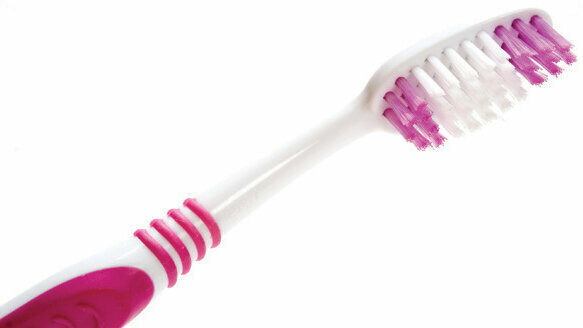This landscape-oriented close-up photograph captures a white toothbrush with striking pink accents. The toothbrush is positioned pointing towards the top right corner, showcasing its design in meticulous detail. The bristles are arranged in an eye-catching pattern with pink at the top and bottom, and a spot of white in the center. The finger pad, designed for a comfortable grip, is a vibrant pink, complemented by additional pink lines accentuating the stem of the toothbrush. The backdrop is a clean, solid white, highlighting the toothbrush as the focal point of this crisp and modern image.